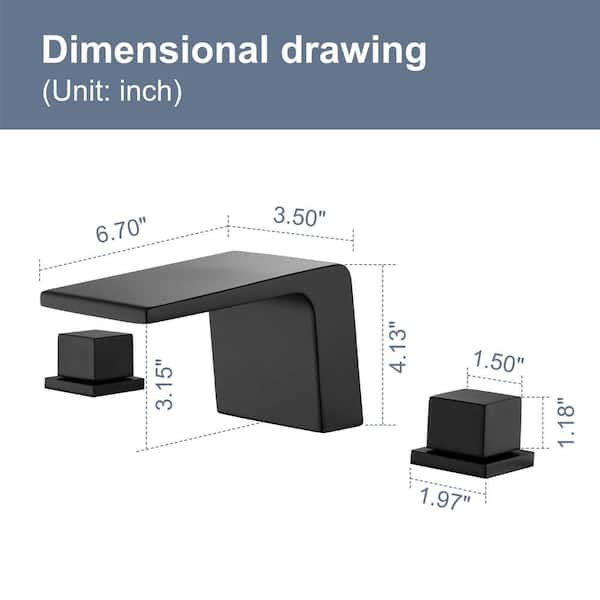This detailed illustration showcases a dimensional drawing with engineering precision. At the top, a gray rectangular banner displays the text "Dimensional Drawing (Unit: Inch)" in white font. Below this header, three intricate diagrams present various components, likely of a bathroom sink faucet. The central figure appears to be the water dispenser, characterized by an extended, diving board-like feature. This piece measures 6.7 inches in length, 3.5 inches in width, stands 4.13 inches tall, and the extension measures 3.15 inches to its tip. Flanking this centerpiece, two identical L-shaped parts are meticulously detailed, with the longest part measuring 6.7 inches marked by a dotted line, and another dotted line indicating a 3.5-inch dimension at the rear. These multiple views collectively provide comprehensive measurements for manufacturing or installation purposes, emphasizing the precise specifications in inches.